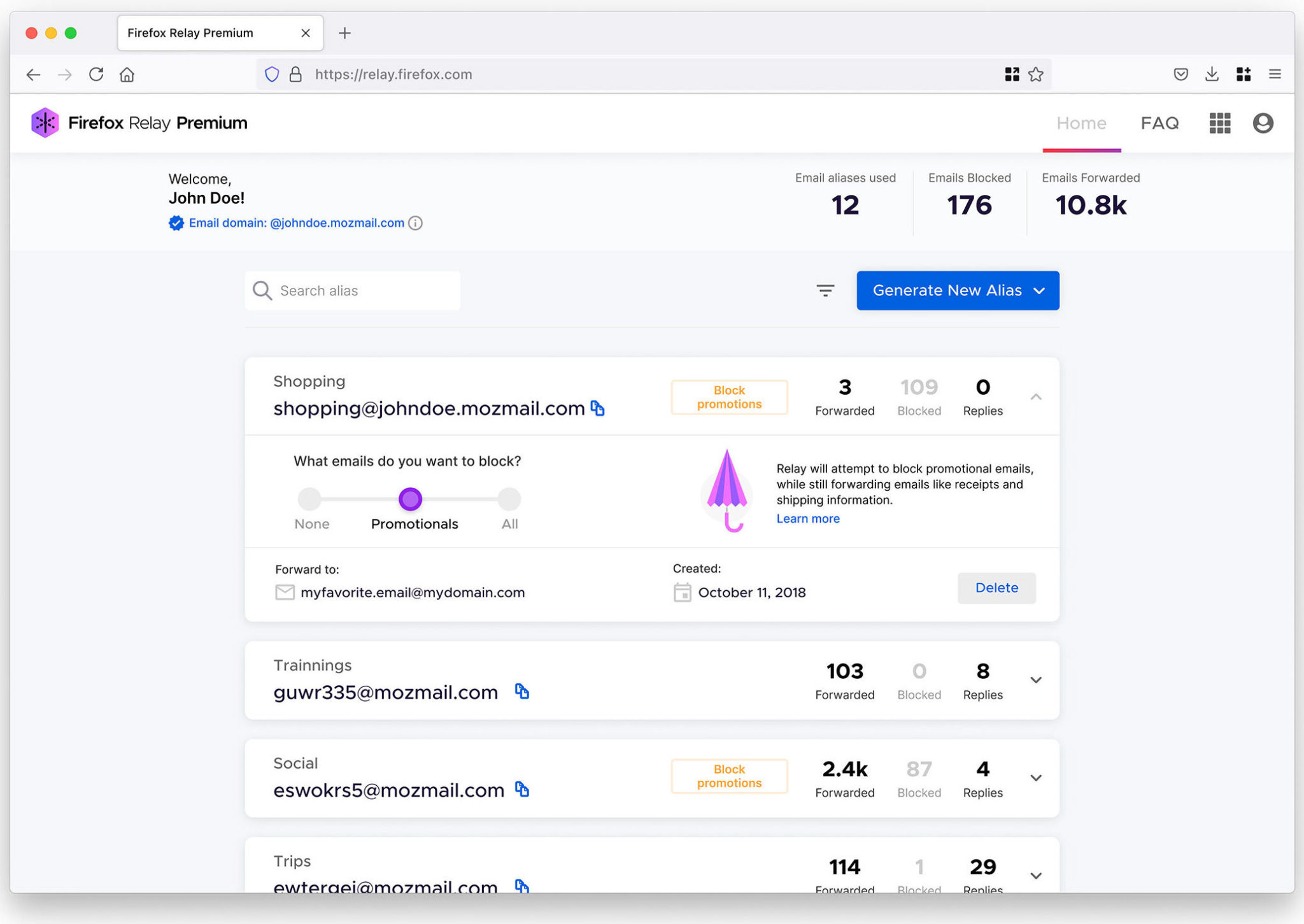Screenshot of a computer screen displaying the Firefox Relay Premium interface. The interface features a light lavender background with darker purple accents. At the top, the text "Welcome John Doe" is prominently displayed. Below, statistics are provided: "Email aliases used: 12," "Emails blocked: 176," and "Emails forwarded: 10,800." Options to "Generate new aliases" are available with a dropdown menu, and a "Search aliases" function is located to the left. The email domain shown is "johndoe.mozmail.com." Additional information about headshopping and training opportunities is listed near the bottom of the screen.